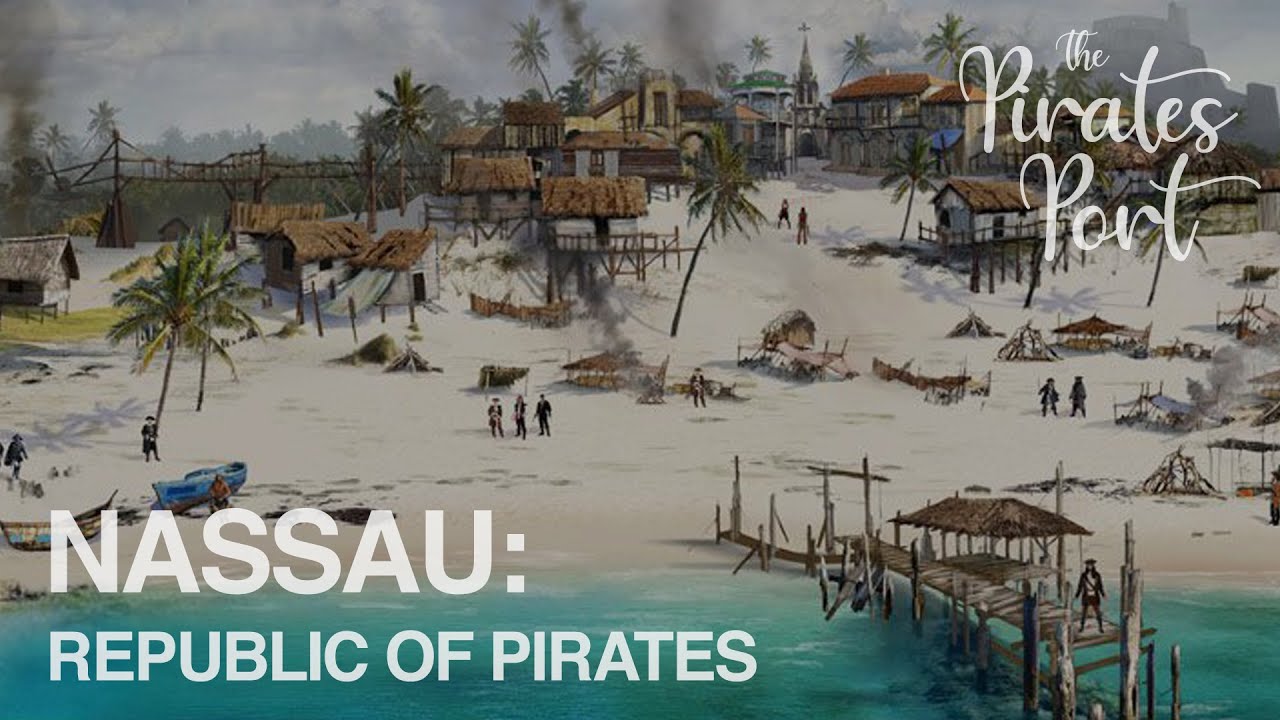The cartoon poster vividly depicts a pirate-dominated scene on a beach, advertising areas of Nassau with the title "Nassau, Republic of Pirates" prominently displayed in the lower left corner and "The Pirates Port" in the upper right. The foreground features a dock extending into light bluish-green water, constructed with sticks or logs and topped with a straw roof. Pirates can be seen standing guard across the beach, suggesting they have taken control of this place. The beach itself is scattered with stranded boats and kayaks, and there are flames from makeshift fires burning. Surrounding the beach are several bamboo-covered huts and palm trees, all leading up to a hillside where more huts rest on stilts, connected by a wooden walk bridge. The background includes additional buildings, likely homes, palm trees, and a hazy atmosphere with cloud cover, adding to the feeling of a lush, tropical pirate haven.